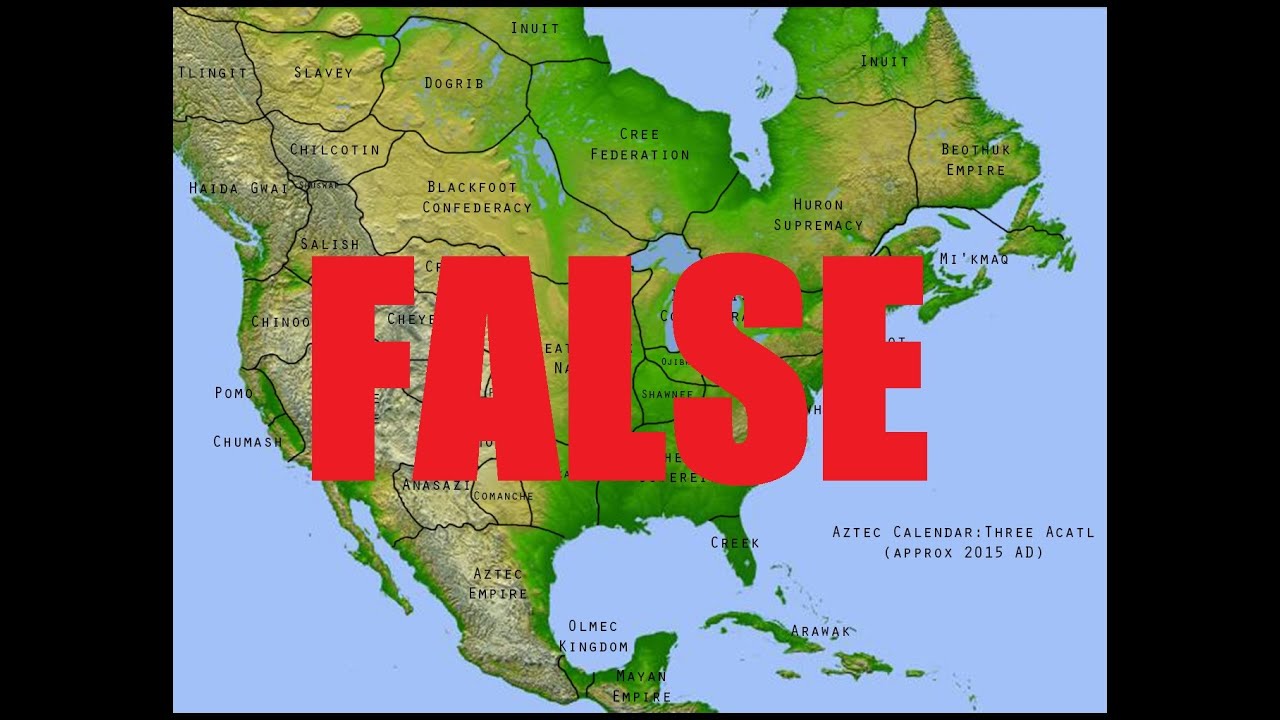This is an illustration of a historical map of North America, featuring the old shapes and outlines of the United States, Canada, Mexico, and some Caribbean islands. The map vividly shows various sections labeled with names of aboriginal tribes and ancient civilizations. At the top, it prominently reads "Inuit," indicating the indigenous people traditionally dwelling in the icy areas. Different sections within the mainland display names such as "Selvi," "Dogi," "Kifa Federation," "Bigfoot Confederation," and more, though some are obscured by a dominant feature of the map.

A significant detail is the large, bold, red text overlaying the center of the map that reads "FALSE," which is the focal point of the image. This bold declaration partially covers other names and sections making them blurry and hard to read. The map is colored with a light blue sea and mainly green landmass.

In the southern parts of the map, it depicts ancient civilizations such as the "Aztec Empire," "Olmec Kingdom," and the "Mayan Empire." In the Caribbean region, islands are labeled with names like "Aramec." Additionally, there is a note at the top labeled "Aztec Calendar 3 A.C.A.T.L., approximately 2015-18," potentially indicating an alternate historical timeline or referencing an ancient dating system.